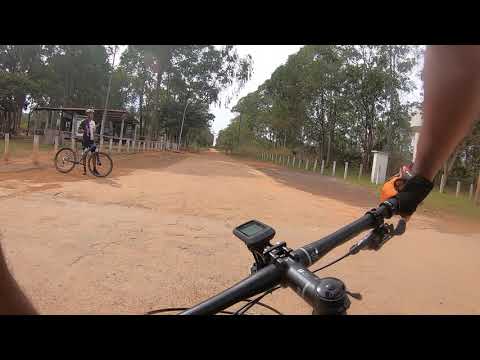This image captures an outdoor scene on a cloudy day from the perspective of someone riding a bicycle, evident by the view over the bike's handlebars and the gloved hand gripping the right handle, which is angled left. The path ahead is a wide, brown dirt trail, extending far into the horizon, flanked by very tall trees with patches of greenery. The trail is also lined with short white posts, approximately two to three feet high. Another cyclist is visible a few feet ahead on the left side, either riding or standing with their bike. In the background, there's a structure resembling a shack or tenement on the left side. The sky above is gray and overcast, adding a muted, ambient light to the scene. A speedometer is noticeable on the handlebars, contributing to the detailed view from what appears to be a GoPro camera.